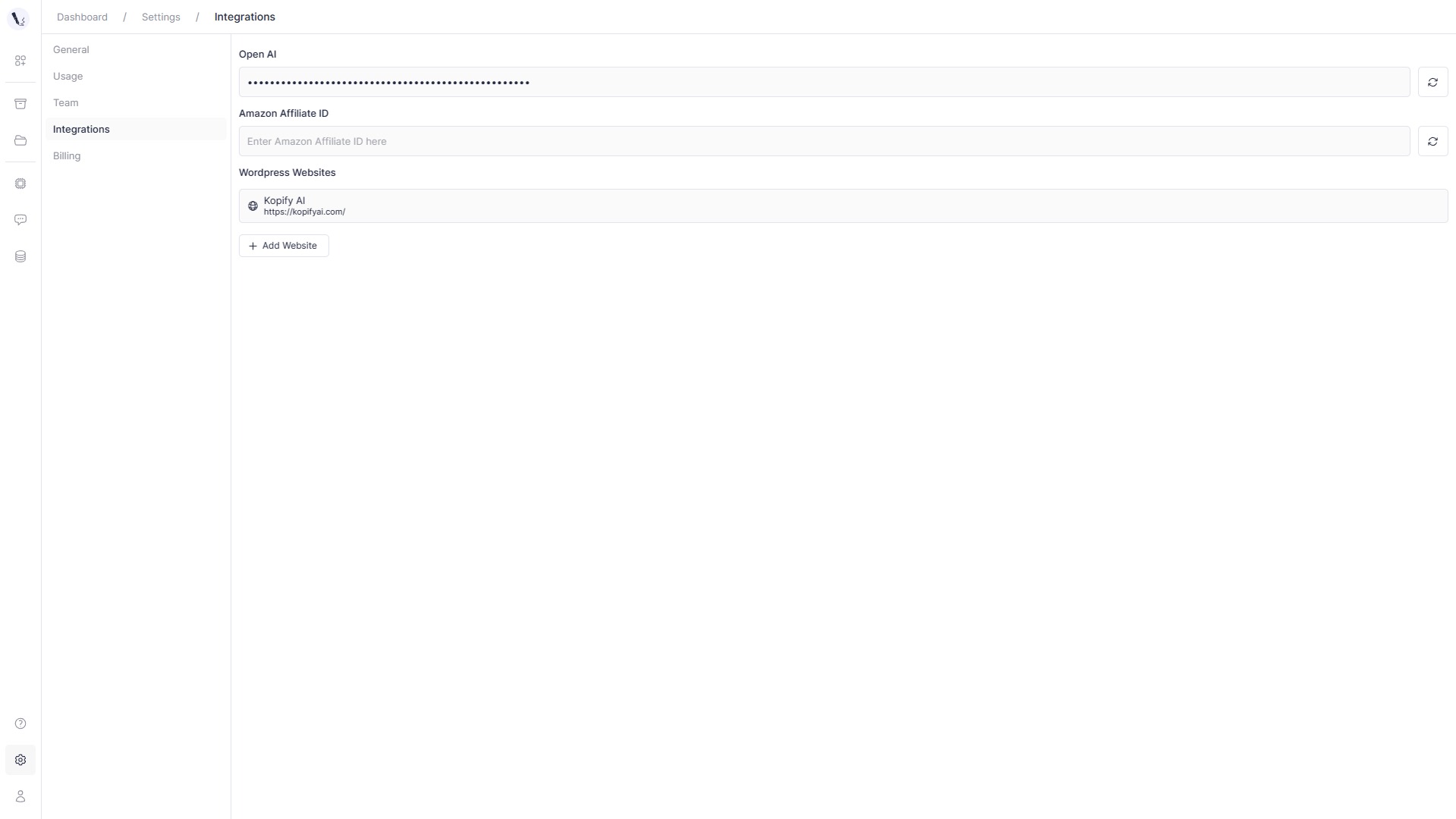Sure! Here is the cleaned-up, detailed description:

The image features a dashboard with a white background. At the top, there are three options labeled "Dashboard," "Settings," and "Integrations," with "Integrations" highlighted in bold black. 

Below that, there is a section that contains labels: "General," "Usage," "Team," and "Integrations," all listed within a small gray box. Next to these, you find another option labeled "Billing."

On the right-hand side of the image, the text "OpenAI" is displayed. There is a field for entering a very long password placed within a gray box. Below this, there is an "Amazon Affiliate ID" section, which includes a prompt to "Enter Amazon Affiliate ID here" within a gray box similar to the password field.

Further down, there’s a section titled "WordPress Websites." In this section, within a gray box, you see a URL "Copify AI HTTPS://copify.com/" followed by options to add more websites. There is also a small box with a gray line around it and a plus sign, labeled "Add Website."

This is the entire layout presented in the screenshot.